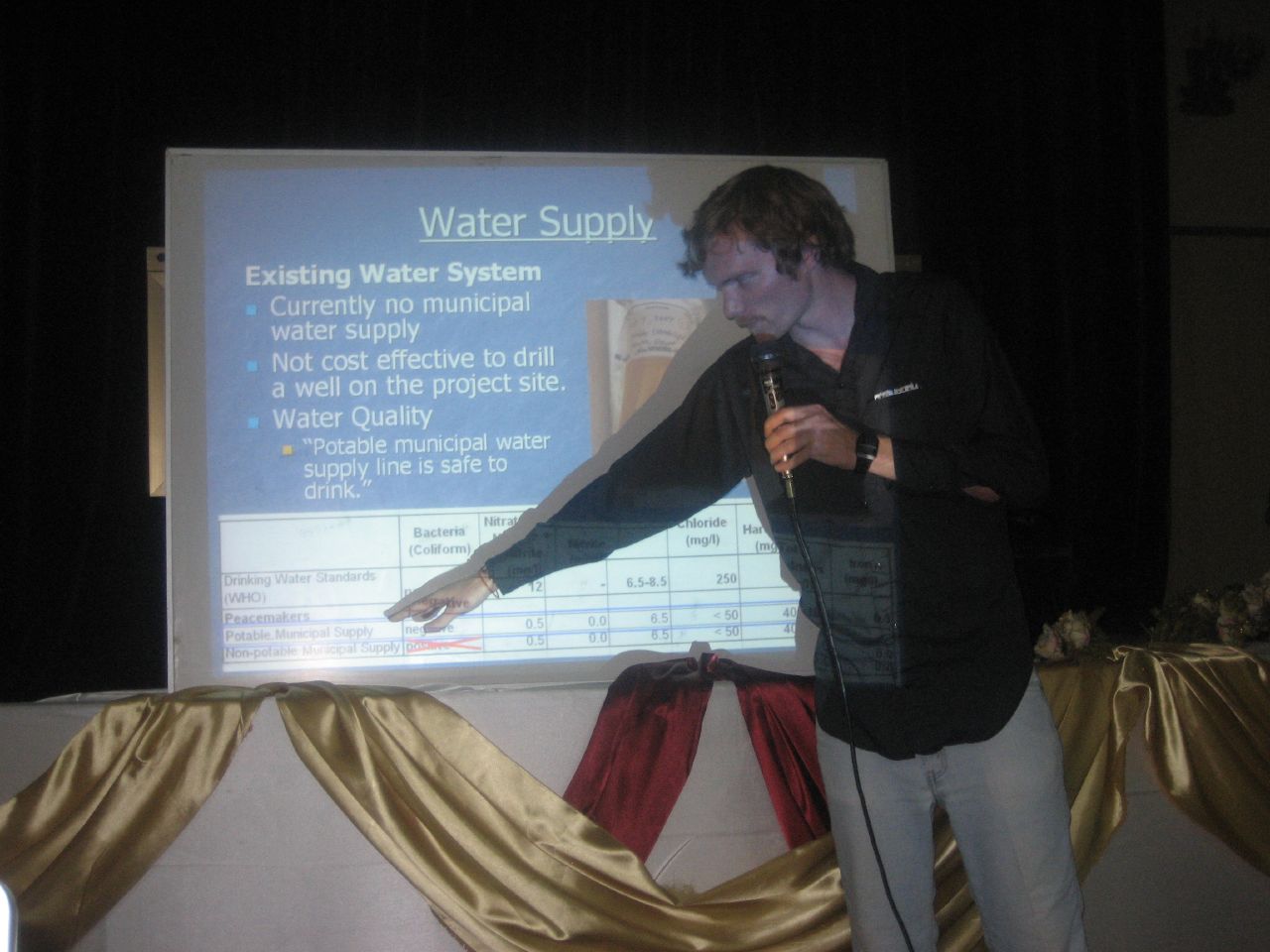In this detailed photograph, a man is presenting in front of a projector screen. He holds a microphone in his left hand, and although his lips are not open, he appears to be in the midst of delivering a presentation. Wearing an untucked black button-down shirt with a possibly white label on the left chest area and gray slacks, he points with his right hand to the lower portion of the screen. The screen displays a slide with bulleted points and a white chart. At the top of the slide, against a blue background, white text reads "Water Supply." Below, key points include: "Existing water system," "Currently no municipal water supply," "Not cost-effective to drill a well on the project site," and "Water quality. Potable municipal water supply line is safe to drink." The screen is situated behind a table draped with elegant gold and burgundy linens that cascade in a V-shape, set against a black backdrop.